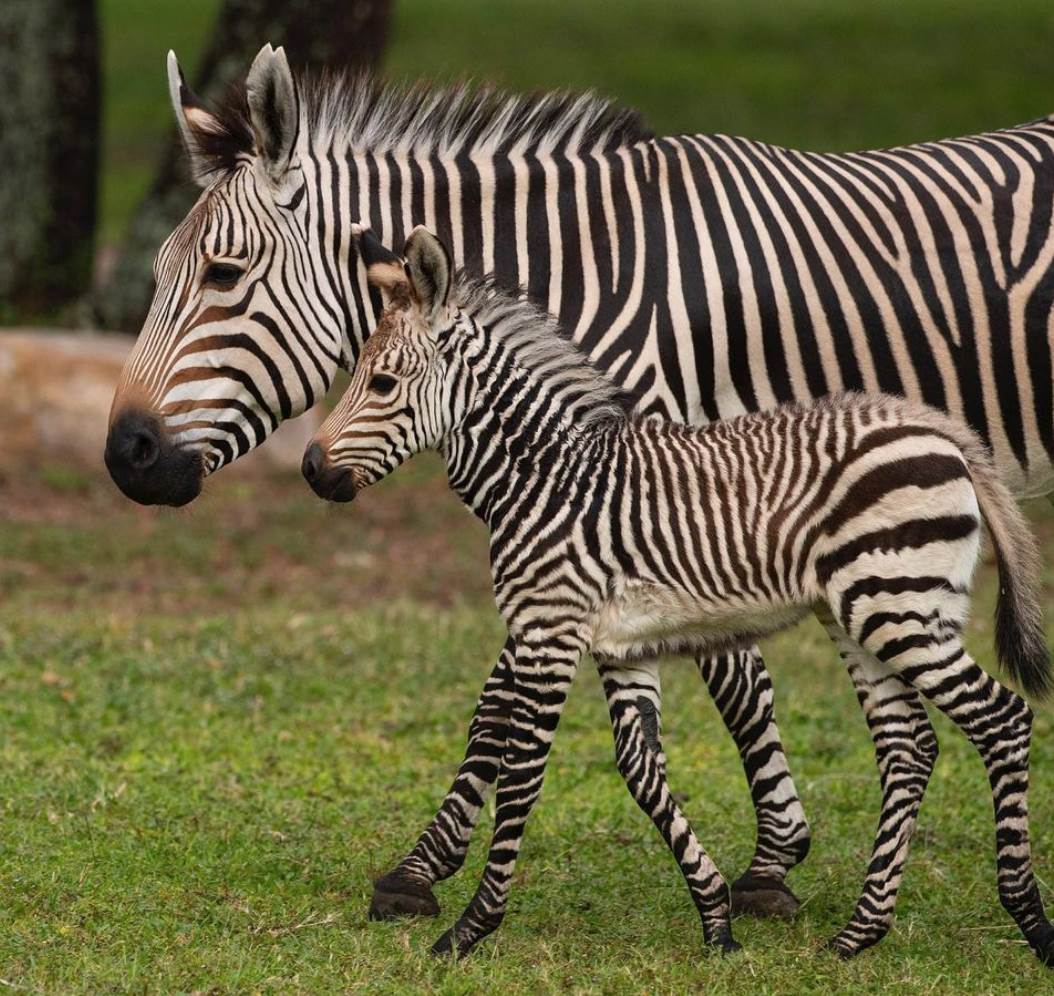The photograph features an adult zebra and its smaller offspring traversing a short, mowed grassy area from right to left. Both zebras, adorned with characteristic black and white stripes and short manes, have ears erect and black muzzles. The adult zebra, fully grown and positioned behind, follows closely behind the juvenile zebra, whose head is about a foot or two lower than that of the adult. The zebras appear relaxed and at ease, suggesting a calm environment. In the blurred background, there are tree trunks and green blurriness indicative of either a zoo setting or the African countryside, with patches of brown adding to the natural ambiance. The zebras exhibit a slightly dusty appearance, giving a lived-in feel to their striking coats. The photograph, presented in a square frame, captures a tender moment of these graceful animals side by side.